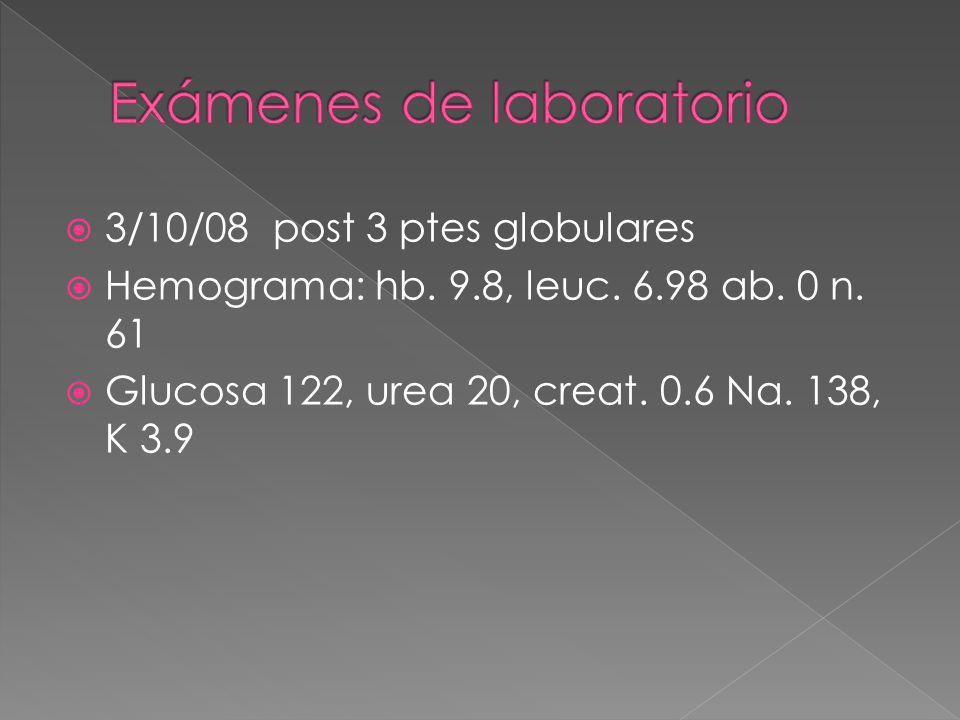The image is a slide presenting laboratory examination results. The background consists of two diagonally divided triangles: the upper right triangle is dark gray, while the lower left triangle is a lighter gray. At the top of the slide, in pinkish-red font, it reads "Exámenes de Laboratorio," which is Spanish for "Laboratory Exams." Below this headline, there are three pink bullet points, each followed by white text displaying the results:

1. The first bullet point starts with the date "3-10-08," followed by "Post 3 PTE globulars."
2. The second bullet point lists "Hemograma HB 9.8," "Leukocyte 6.98," and "AB 0N61."
3. The third bullet point provides the measurements "Glucosa 122," "Urea 20," "Creat 0.6," "Na 138," and "K 3.9."

The entire slide appears to be part of a medical presentation or report, showcasing laboratory test results in a structured and visually distinct format with the gray background and vivid pink elements for emphasis.